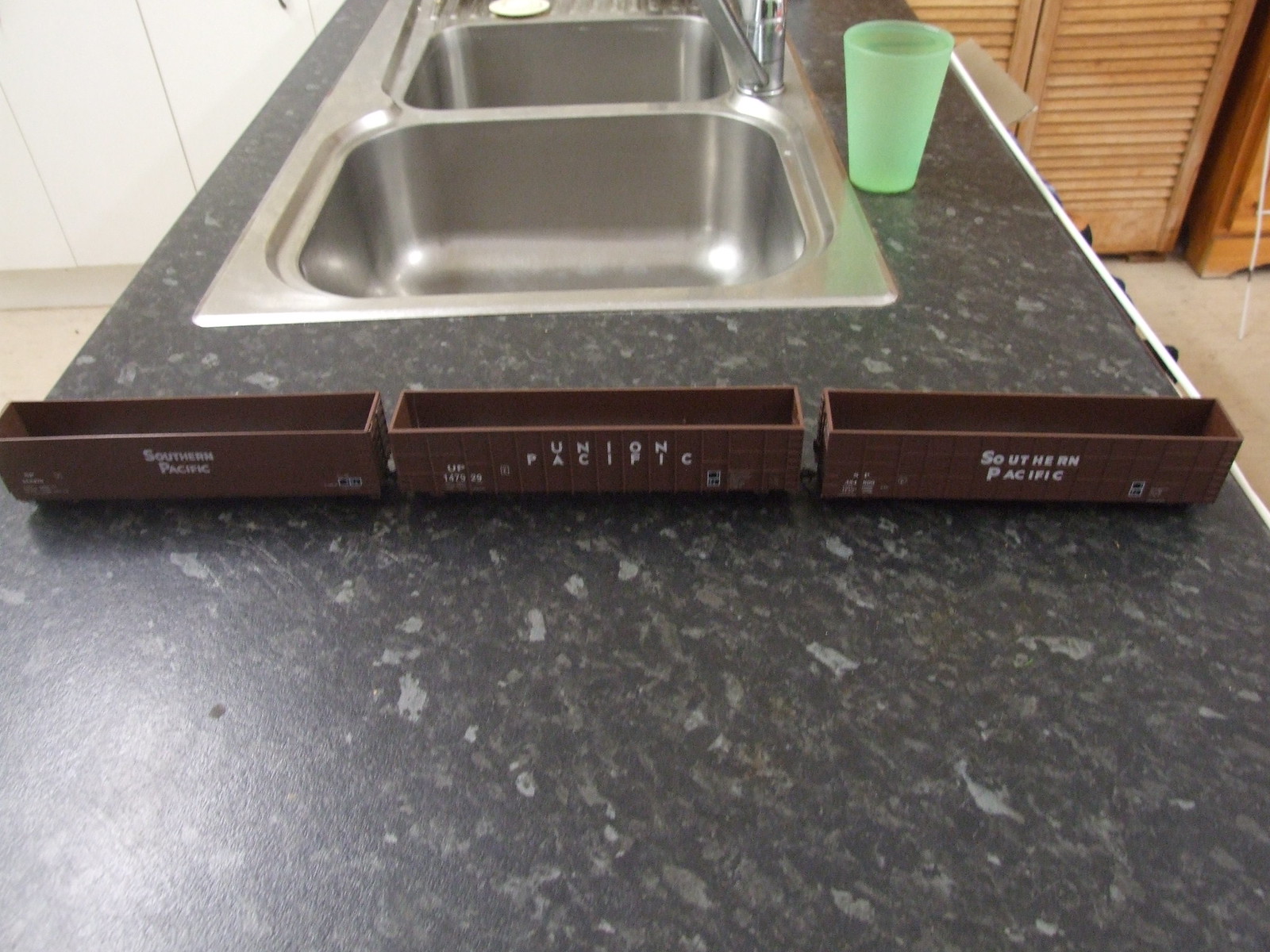The image depicts a spacious kitchen counter, likely crafted from gray and white marble, stretching approximately five to six feet long. Prominently displayed on the counter are three toy train cars, each around 8 to 10 inches in length and brown in color with white lettering. The central train car is labeled "Union Pacific," while the two flanking it are marked "Southern Pacific." These toy cars appear to be parts of a child's playset, designed to resemble trailers that might carry coal or wood. Positioned behind the toy trains is a dual-compartment stainless steel sink, with a light green glass, about 7 to 8 inches tall, situated adjacent to it. In the background, brown-colored cabinets can be seen, and the floor beneath is a very light brown shade. The detailed depiction of the train cars, marked with their respective railroad names, stands out as the most striking and central feature of the scene.